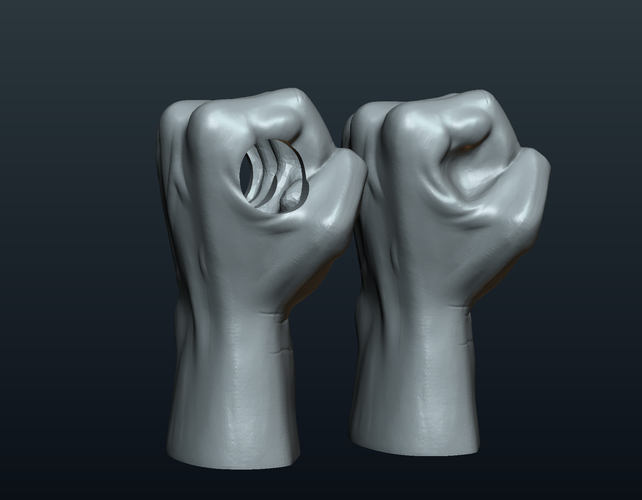The image features two 3D-rendered sculptures of human fists, prominently displayed against a dark, gradient background that shifts between black and dark gray. Both fists are positioned side by side and oriented upside down, extending approximately three to four inches past the wrist. Each fist has meticulous detailing that showcases musculature, veins, and wrinkles near the wrist, conveying a realistic texture despite their overall light gray or dark silver coloring.

The fists differ in one significant way: the fist on the left has a large, visible hole that pierces straight through its center, while the fist on the right is fully enclosed, with its thumb extended outward. The surfaces of both sculptures are somewhat shiny, emphasizing their stone-like material appearance, reminiscent of objects that could be either 3D-printed models or carved out of stone. The overall impression is that of an art piece, with both fists serving as evocative symbols, standing resolutely in the center of the composition.